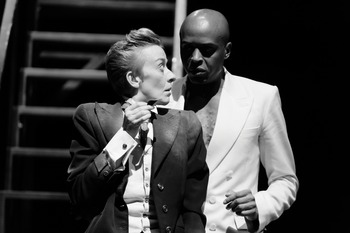This detailed black and white photograph depicts a dramatic scene featuring a black man and a white woman, possibly mid-performance. The background is stark black with a staircase or ladder situated behind them, adding a sense of depth to the image. The man, placed slightly behind and to the right, has a bald head and broad nose, and is wearing a white blazer without a shirt, drawing attention to his bold appearance. The woman, positioned slightly in front and to the left, has a Caucasian complexion with short, gelled-up hair that adds a dynamic flair to her androgynous features. She is dressed in a black blazer with pronounced shoulder pads over a button-down shirt with French cuffs. Her body is turned sharply to the right as she looks back at the man with a surprised or inquisitive expression. She has her right hand raised, and his hand is reaching towards her, indicating a moment of intense interaction or communication between the two characters.